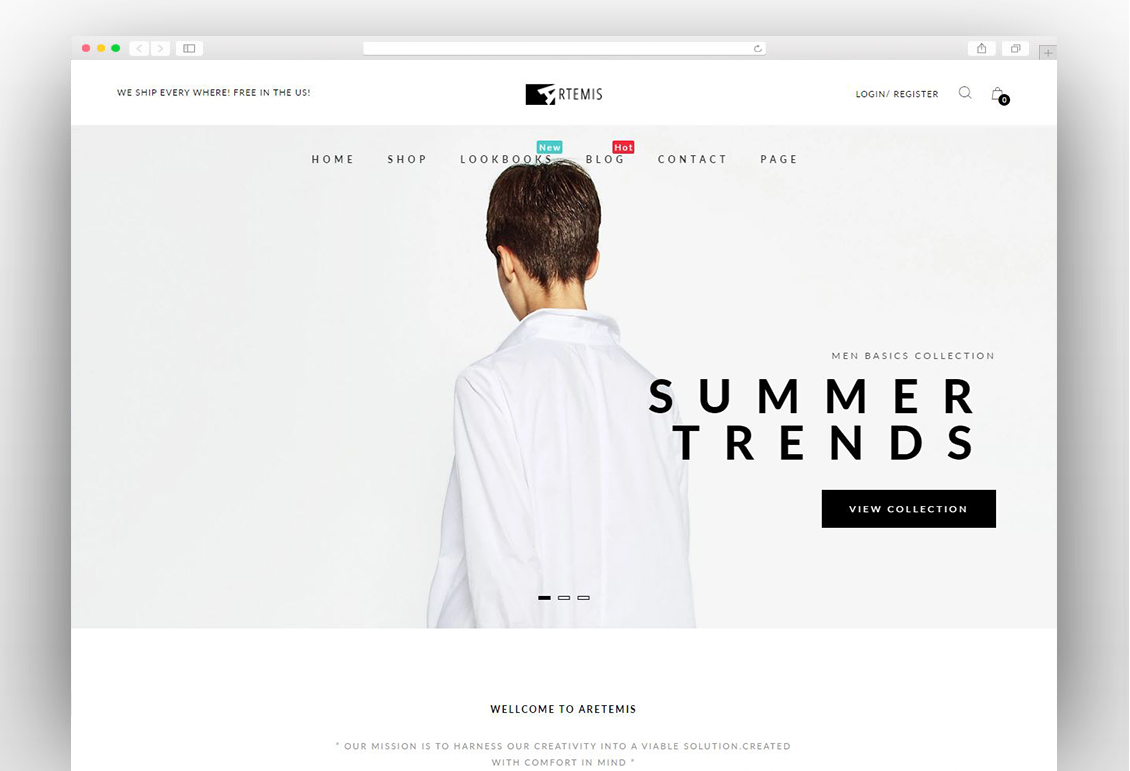This is a detailed caption for the described image:

---

The webpage presents a sleek design with a light gray border spanning the top and sides, about an inch in width. Within this boundary, an even lighter gray header stretches across the top. On the top left corner of this header, there are three small circles colored red, yellow, and green respectively, followed by two squares—one containing a left-pointing greater than symbol and another with a right-pointing one—and an additional square with just a simple outline. Centered within this header lies a prominent search bar.

Further to the top right, there are two more squares containing different icons. Beneath the search bar, a one-inch white border separates elements. To the right side of the border, there's an account option labeled "Login/Register". Adjacent to this, a search icon and a bell icon are positioned, the latter marked with a black circle indicating eight notifications. To the left of this area, a statement reads, "We ship everywhere free in the US".

Below this section sits a captivating image against a light blue background, depicting a person with short black hair and a white long-sleeve shirt. Positioned above their head are two tabs: a blue tab with the word "NEW" inscribed in white, and a red tab labeled "HOT". Above these tabs lies a navigational menu with options: Home, Shop, Lookbooks, Blog, Contact, and Pages.

To the individual's right shoulder, bold black capital letters announce "SUMMER TRENDS," while above this, a subtitle reads "Men's Basics Collection". Below, a black tab with white lettering invites visitors to "View Collection".

Around this central image and information section, a two-inch white border frames the webpage content. In the center of this border, the greeting "Welcome to Artemis" is displayed, albeit with an unusual spelling featuring an extra "L" in "Welcome". Below this greeting, two lines of additional information are provided.

---